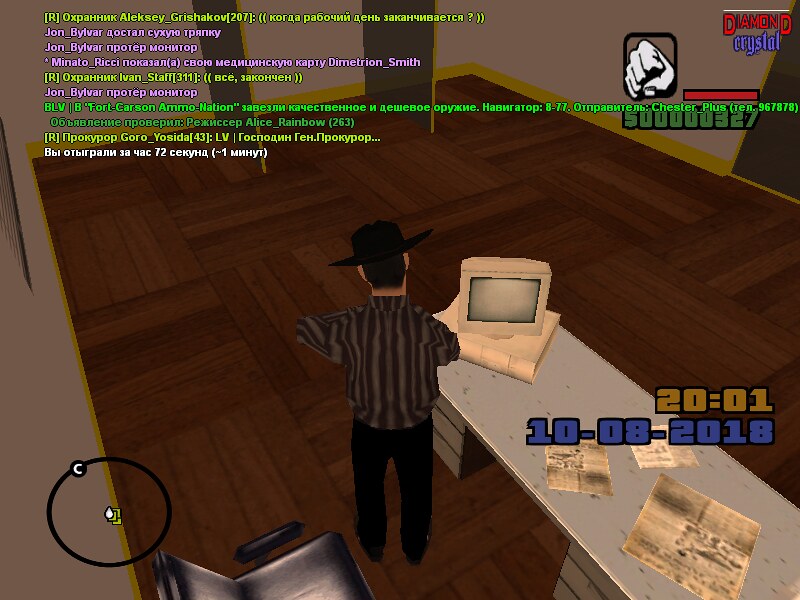In this detailed, pixelated image from a Grand Theft Auto game, we observe a man standing in an office setting, in front of a computer with an inactive screen. The character, dressed in a striped shirt, black pants, and a distinctive black cowboy hat, has short hair and stands beside a white desk cluttered with newspaper clippings. The computer tower is positioned beneath the monitor, and the table it rests on appears dirty. The floor beneath them looks like it has a wooden texture. Important text elements include a date displayed as "2001" and "10-08-2018" in blue. The game's interface reveals at the top right a fist holding money, indicating a balance of $327, alongside a red bar. A chat box with Russian text is visible at the top left, while a map interface sits at the bottom of the screen.